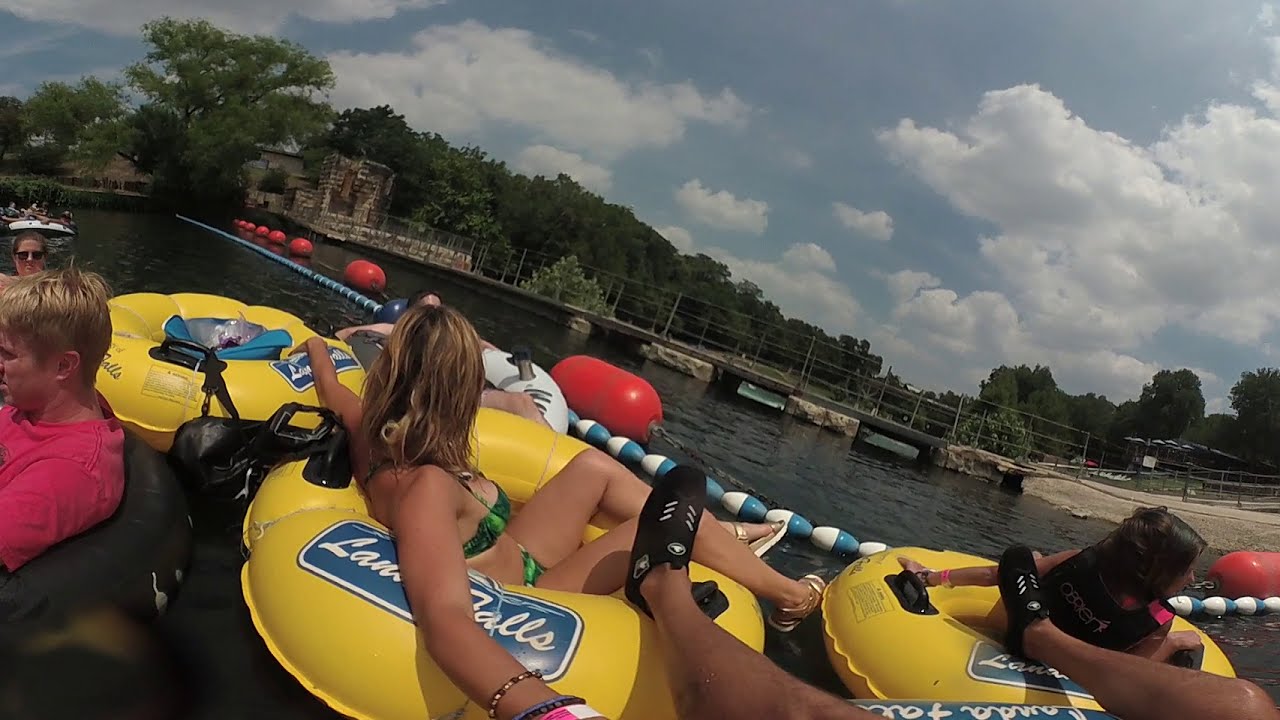A vibrant scene at a water park showcases several people floating on yellow inner tubes in a leisurely river with a strong current. Dominating the center of the image is a girl in a green bikini, her light brown shoulder-length hair facing backward as she extends her arms outward and leans back in her float. Her gold-colored sandals add a touch of shimmer as her legs protrude towards the right, just above the water.

To the right is another participant, partially visible with legs extending from the knees down, sporting black shoes with white stripes. One foot rests on the girl's inner tube while the other is positioned on an adjacent tube housing another person. Nearby, a woman with dark black hair, turning her face towards the bottom right corner, steadies herself on the float.

An empty inner tube floats to the left of the central girl, while behind her sits a man in a pink shirt with blondish light brown hair. Over his head, another figure with sunglasses lurks in the background. Bright blue and white floating cones form a barrier in the water while linked orange cylinders float on the surface as additional dividers.

The water surrounding them is a dark green, gently rippling under a hazy sky filled with a mix of white and gray clouds interspersed with patches of blue. In the background, thick, tall rows of green trees line the edge of the scene, obscured by a fence. Additionally, a stone bridge stretches left and right across the river, and the yellow inner tubes, adorned with black handles, feature branding in cursive white text on blue rectangular bubbles. Red oval markers at regular intervals reinforce the boundaries of the water space, contributing to a lively, contained atmosphere where people enjoy the tranquil float.